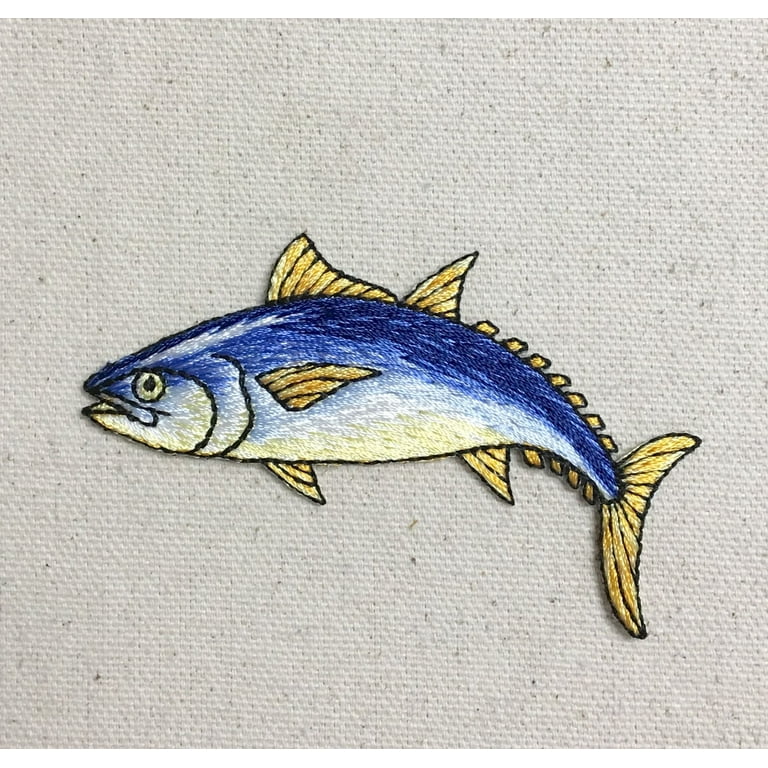The image showcases an intricately embroidered patch of a vibrant fish, positioned on a textured, off-white, speckled material, possibly canvas or a tan-colored fabric such as a shirt. The fish, stitched with remarkable detail, features a striking combination of blue and white on its body, with a white belly and a blue top. Its bold black outlines accentuate its detailed features, including its gills and multiple fins. Notably, the fish has a yellow eye, and its fins and tail are a vivid yellow, with seven small yellow fins trailing from its back to its tail. The design boasts a 3D effect, suggesting a complex overlapping stitching technique, distinguishing it from simpler needlepoint designs. The fish, viewed in profile and facing left, appears almost lifelike with highlighted shadows underneath, enhancing its dimensionality.